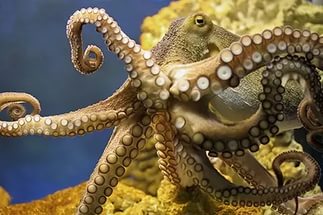The image is a stunning underwater photograph showcasing a small octopus centrally positioned against a beautifully clear, deep blue ocean backdrop. In the foreground, the octopus's brownish-tan tentacles extend in all directions, spiraling at the ends, and are adorned with rows of shiny, white suckers that resemble tiny pearls. The head of the octopus is a brownish-spotted color, with its left eye prominently visible, giving the impression that it's peering directly at the camera, which adds a slightly eerie effect. In the background, the ocean floor is visible with hints of brown and yellow, possibly indicating a coral reef or similar underwater landscape. The image is remarkably clear and detailed, allowing for a vivid depiction of the octopus and its environment.